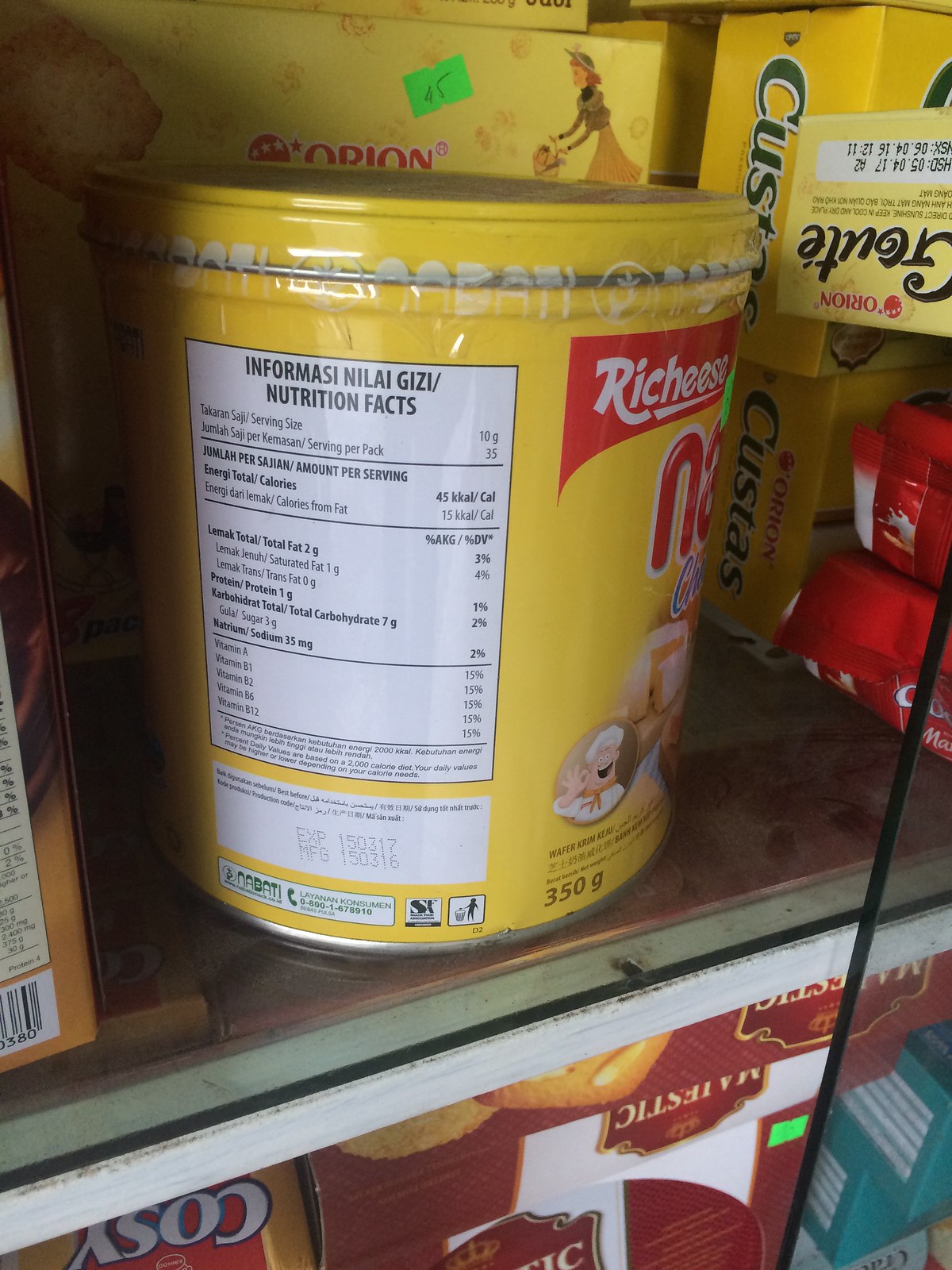This image depicts the nutritional facts label of a baby food powder, specifically formulated for mixing with milk. The label details the various vitamins and nutrients included in the product, such as Vitamin K, Vitamin B2 (Riboflavin), Vitamin B3 (Niacin), and Vitamin B12. The inclusion of these essential vitamins indicates the product's role in supporting the healthy development of infants. The detailed nutritional information provides parents with the reassurance of the product’s nutritional benefits.